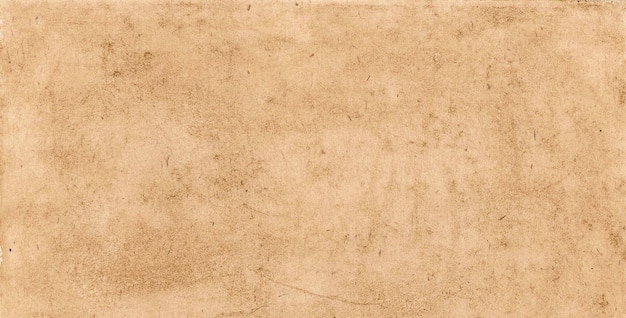The image depicts a plain, textured background that completely fills the frame. The primary color of the background is a range of beige and brown tones, including shades of tan, light brown, dark brown, and off-white. The surface appears rough and uneven, with several dark marks, spots, and splotches scattered throughout, resembling characteristic imperfections found in old film or photographs. Notable features include a curvy line positioned towards the bottom middle of the background and areas of discoloration and fading, most prominently on the left and right sides. Despite these details, the image contains no discernible objects, text, or patterns, leaving the focus solely on the unique and varied textures and colors of the background itself.